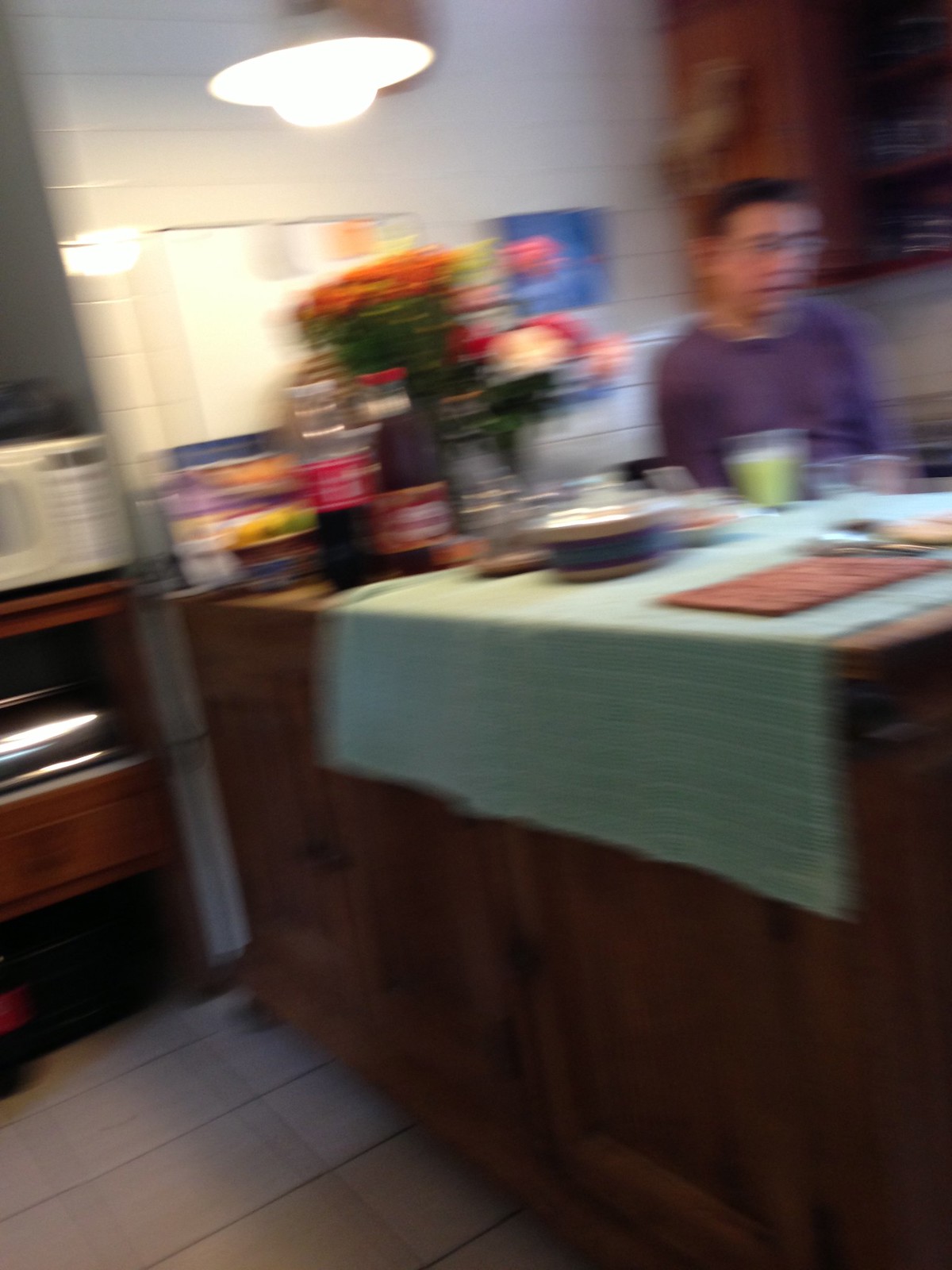This vertical, blurry color snapshot captures a cluttered kitchen scene centered around a wide counter extending from a white tiled wall, rather than an island. The counter holds a mix of everyday items, including a place setting with utensils, placemats, possibly a bottle of Coke, and a vase with flowers. At the edge of the counter, draped with a long towel, sits an Asian male with short hair and glasses, wearing a purple shirt. He is drinking something green from a glass. There is a hint of a bottle of Coke and possibly some butter nearby. Behind him, pine wooden cabinets and a small white microwave partially visible, further enhance the kitchen ambiance. The beige-tiled floor and a hanging ceiling light, which contributes to the blurriness, complete the setting. A calendar or whiteboard is discernible on the wall behind, adding a touch of personal detail to the scene, which captures a moment of everyday life amidst the bustling kitchen environment.